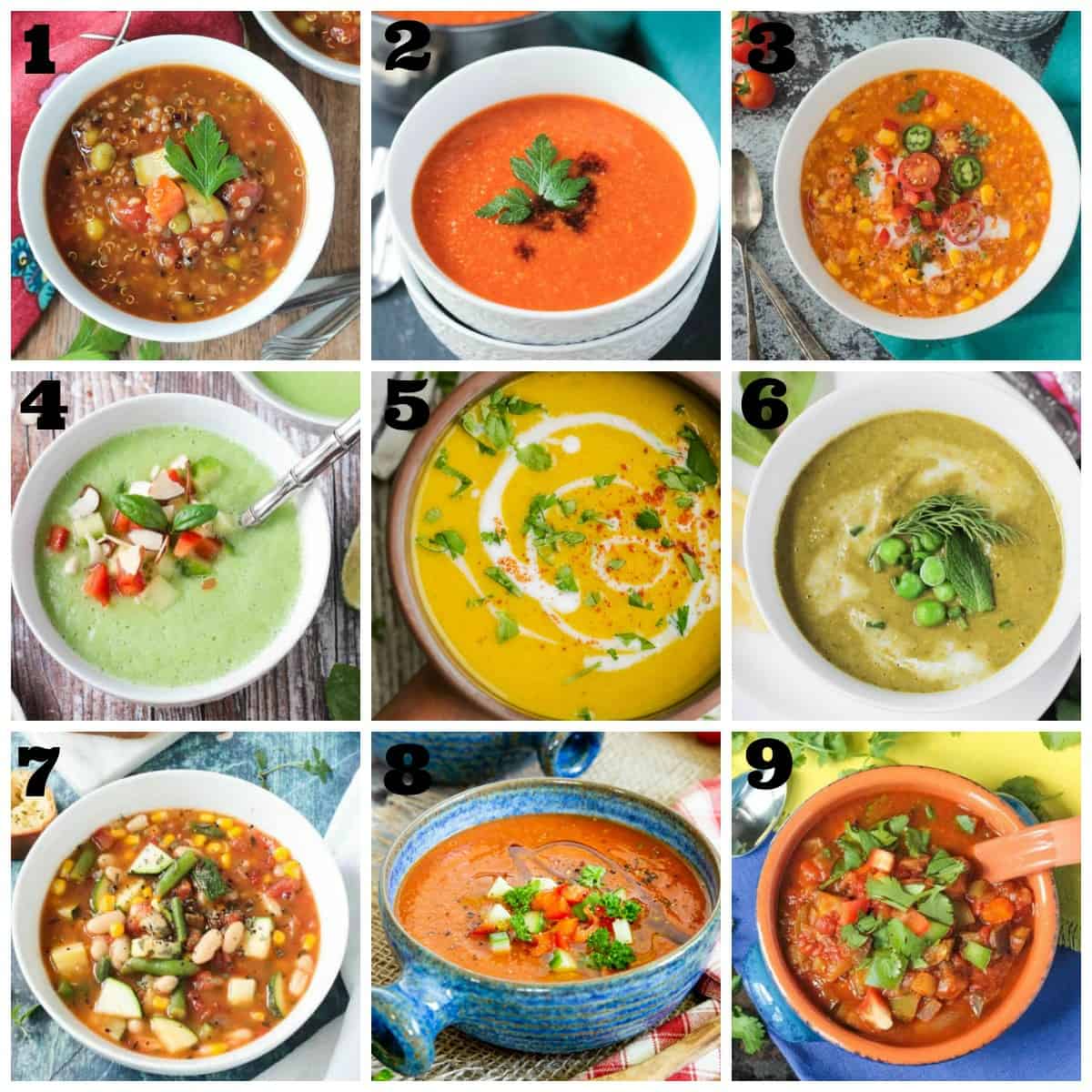The image is a detailed collage featuring nine distinct photographs of different types of soups, arranged in a three-by-three grid of square photos. Each square is numbered in the upper left corner with solid black numerals, ranging from one to nine, starting from the top left corner and ending at the bottom right. The soups are presented in a variety of bowls, including white and blue ones, and each bowl contains a unique type of soup showcasing a rich array of colors and ingredients. 

- **Top Row**: 
  - **Box 1 (top-left, number one)**: Brown soup with a variety of ingredients, including beans. 
  - **Box 2 (top-middle, number two)**: Classic tomato soup.
  - **Box 3 (top-right, number three)**: Orange soup featuring peppers and corn, potentially rich in vegetables.

- **Middle Row**: 
  - **Box 4 (middle-left, number four)**: Mint green soup, likely gazpacho, containing ingredients like tomatoes and onions. 
  - **Box 5 (center, number five)**: Bright orange butternut squash soup with a cream swirl. 
  - **Box 6 (middle-right, number six)**: Green split pea soup, topped with peas.

- **Bottom Row**:
  - **Box 7 (bottom-left, number seven)**: Red soup with a mix of corn, beans, and other vegetables.
  - **Box 8 (bottom-middle, number eight)**: Another type of tomato-based soup.
  - **Box 9 (bottom-right, number nine)**: Red vegetable soup, containing a variety of vegetables.

Throughout the grid, you'll notice vibrant colors such as reds, greens, and oranges, accentuated by ingredients like tomatoes, peppers, corn, beans, and carrots. Each bowl of soup captures the essence of different flavors and textures, making the entire collage a visually appealing representation of diverse soups.